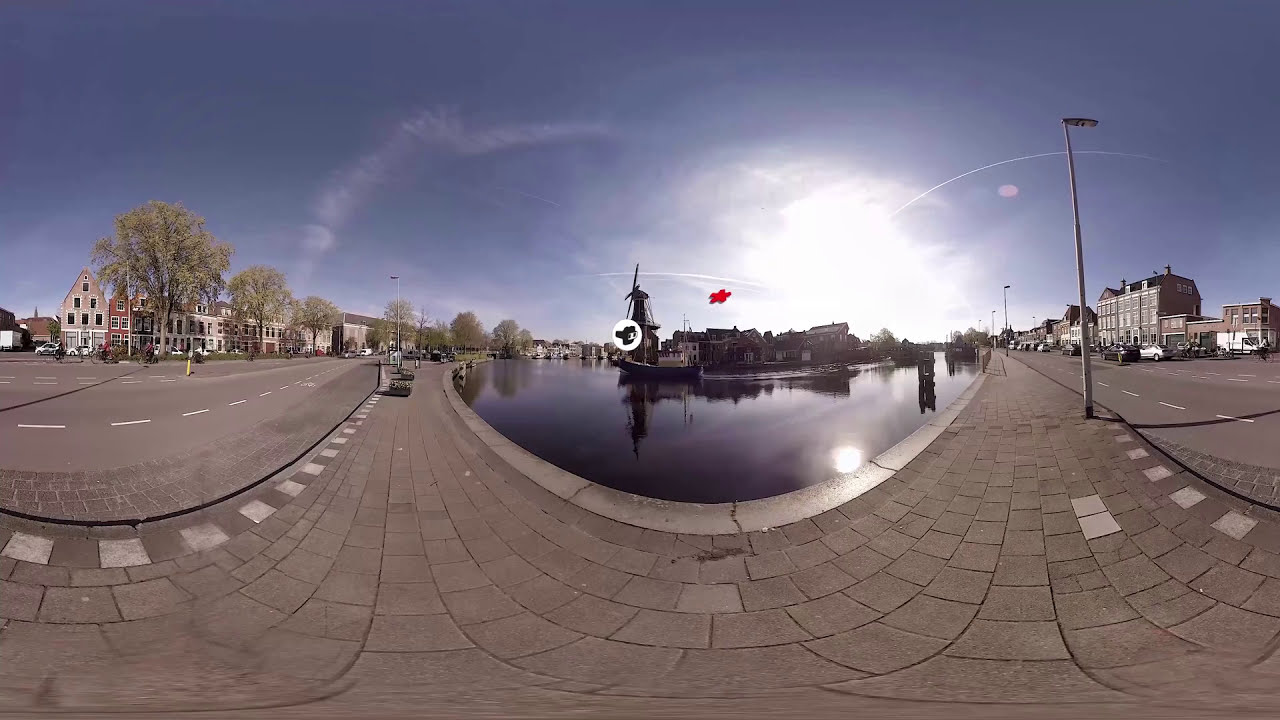The image depicts a horizontally aligned rectangular scene with a clear blue sky and a few feathery white clouds. In the middle of the sky, there's a bright patch of white light. The center of the picture features a small body of water, which appears to be a canal or waterway. This waterway is flanked by sidewalks and streets on both sides. The left-hand side showcases several multi-story buildings adorned with green trees and framed with pointed roofs. These buildings include houses in yellow, red, orange, and white, designed in an A-frame style. On the right-hand side are more boxy, multi-story buildings, likely storefronts or commercial structures, in shades of gray. Among these buildings, there's a lamppost standing by the paved street. The street on the right has at least three or four lanes, dotted cars, and extends into the background where more multi-story buildings are visible. Additionally, a bright red floating object is seen above a cluster of the right-side buildings. In the very center of the waterway, there's a notable statue and a windmill with a red flag. The entire paved area is primarily gray-bricked with a blend of white dotted lines marking the road and walkways. The overall scene is daylight illuminated, casting a beautiful light across the area.